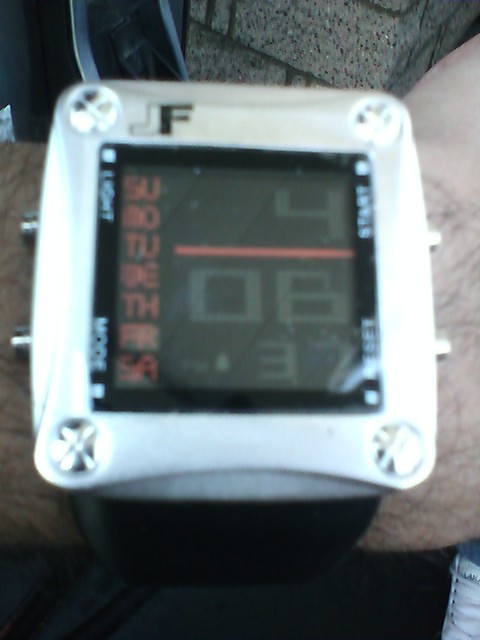The image is a close-up of a white, cube-shaped electronic device resembling a portable game box or wristwatch, but it is confirmed to be a clock. The clock has a black screen displaying numbers and possibly abbreviations in red. The screen shows various details such as "Sunday, Monday, Tuesday, Wednesday, Thursday, Friday, Saturday" along the side, indicating weekdays, and numerical readings of "4," a red line, "06," and "37," likely representing the time 4:06 and 37 seconds. The device bears the initials "JF." It features four silver buttons or screws, one on each corner, with additional silver buttons situated along the left and right sides. Two flat gray wires extend from the top left of the clock. The device is resting on a curved wooden surface, with a concrete block visible in the upper right background. The photograph also captures a hairy arm or leg nearby, implying the possibility of the device being worn, though it's primarily shown as an object placed on a counter.